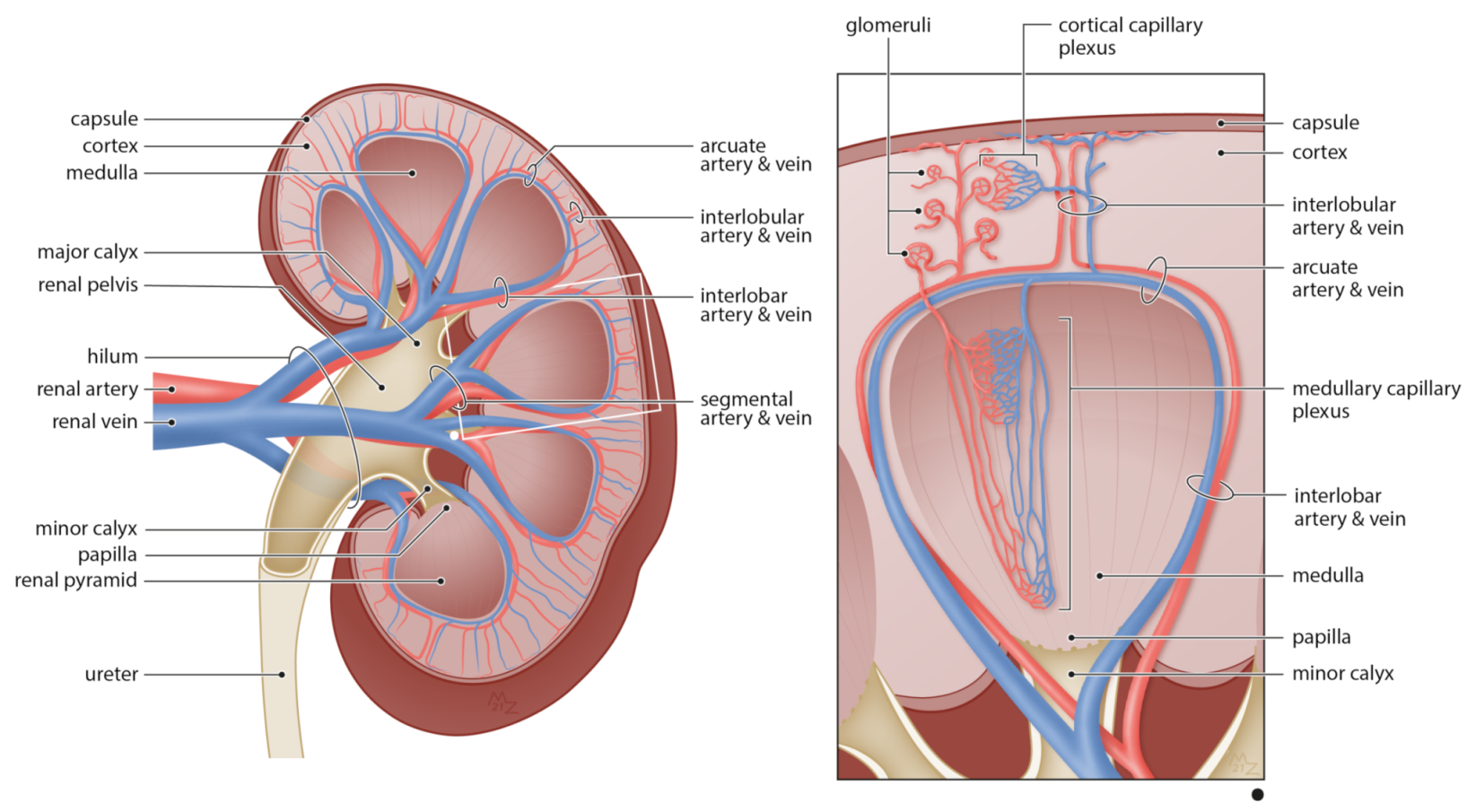The image consists of two side-by-side illustrations set against a white background, resembling a medical journal or presentation. The left illustration is a detailed cross-sectional diagram of a kidney, with reddish-brown borders and various anatomical features labeled in black. This includes the cortex, medulla, pelvis area, renal artery and vein, and the urethra running from the kidney out of the body. The internal structures are vividly depicted, with blue veins and red arteries prominently shown.

The right illustration is a zoomed-in, rectangular section of the kidney, bordered in black, offering a closer view of specific parts such as the cortex, capsule, articulate artery and vein, and medulla. Similar to the left image, this detailed view also uses blue and red to denote veins and arteries, respectively. The inner portion of this close-up is pink, highlighting the intricate network within the kidney. Additionally, the connection between the urethra and the kidney is clearly depicted, along with a small black dot located at the bottom right corner of the illustration.